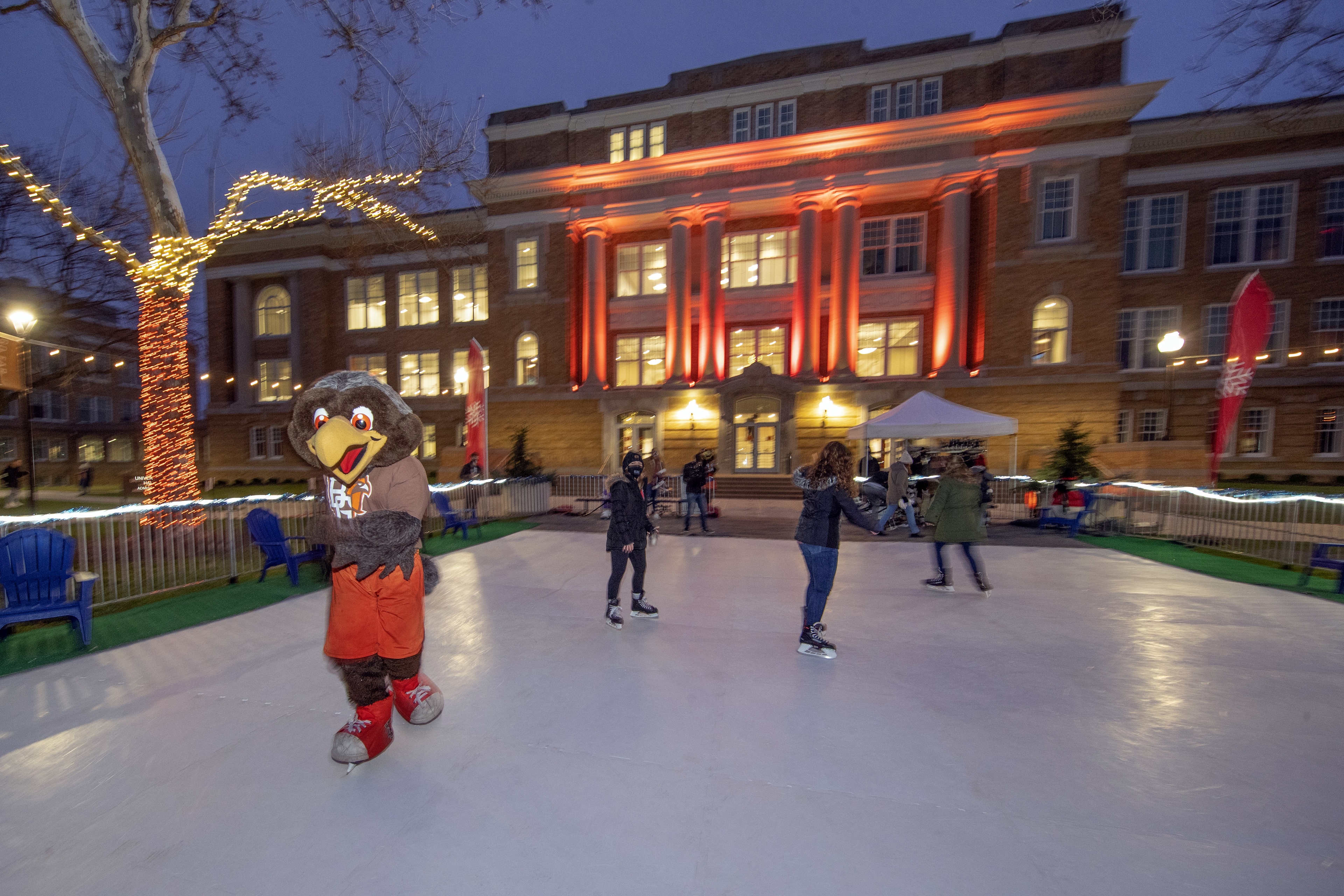The photograph, taken outside at night, captures a lively scene in front of what appears to be a large, multi-story college campus building adorned with numerous windows and illuminated with red and orange lights highlighting its grand pillars. To the left of the image stands a bare tree, decorated halfway up with glowing Christmas lights in shades of orange, gold, red, and white. In the center of the scene is a makeshift ice skating rink set on the grass, bordered by blue chairs. The rink is buzzing with activity as multiple people skate across its surface. Notably, among the skaters is a bird mascot, sporting a brown shirt and orange shorts, resembling an eagle, adding a festive touch to the event. This spirited gathering suggests a special occasion, likely organized by the college, creating a warm and communal holiday atmosphere.